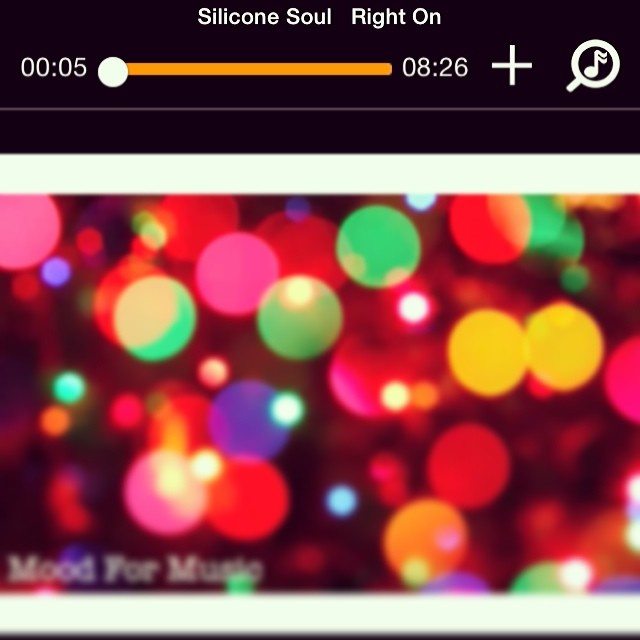This image appears to be a screenshot from a mobile device or music player interface. It prominently features a design of colorful, out-of-focus circles reminiscent of bokeh-style photography, resembling Christmas lights, scattered in various sizes and hues, including black, white, orange, gray, pink, purple, green, tan, white, and yellow. 

At the top of the image, a black bar contains small white text that reads "Silicone Soul Right On," accompanied by a track scrubber with a yellow bar indicating that the track is 5 seconds into an 8-minute and 20-second duration. Adjacent to the track length is a plus sign and a magnifying glass icon with a musical note inside. 

In the bottom left corner of the image, blurry text reads "Mood for Music," further integrating with the vibrant background, making the overall design visually engaging and dynamic.